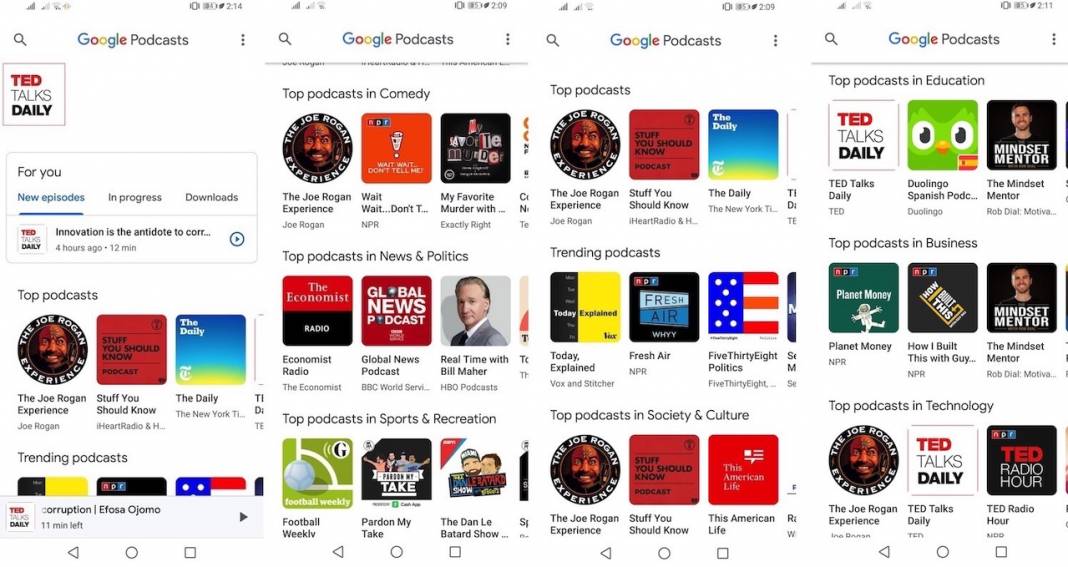This is a screenshot of a Google Podcasts interface on a computer screen, showcasing a range of podcast options in a neatly organized grid. The layout consists of four vertical columns, each displaying various podcasts represented by colorful thumbnails, similar to book covers. 

- At the top of each column, the label "Google Podcasts" is visible. 
- The first column is titled "For You" with clickable options like "New episodes," highlighted in blue, and "In progress" and "Downloads" listed beside it. Featured podcasts include:
  - "TED Talks Daily"
  - Popular selections under "Top podcasts," such as "The Joe Rogan Experience," "Stuff You Should Know," and "The Daily." 
- Details of these shows are clear:
  - "The Joe Rogan Experience" has a black circular icon featuring a bearded man with a wild expression.
  - "Stuff You Should Know" sports a red background with straightforward black text.
  - "The Daily" features an image of a blue sky transitioning to green and yellow hues at the bottom.

- The second column highlights "Top podcasts in Comedy," including:
  - "The Joe Rogan Experience"
  - "Wait Wait… Don't Tell Me!"
  - "My Favorite Murder," partially obscured.

- The third column is labeled "Top podcasts," showing a variety of other trending shows.
- The fourth column is dedicated to "Top podcasts in Education," though specific show details are not mentioned.

This interface allows users to navigate through different genres and categories efficiently, providing vivid visual cues and easy access to popular and recommended podcasts.